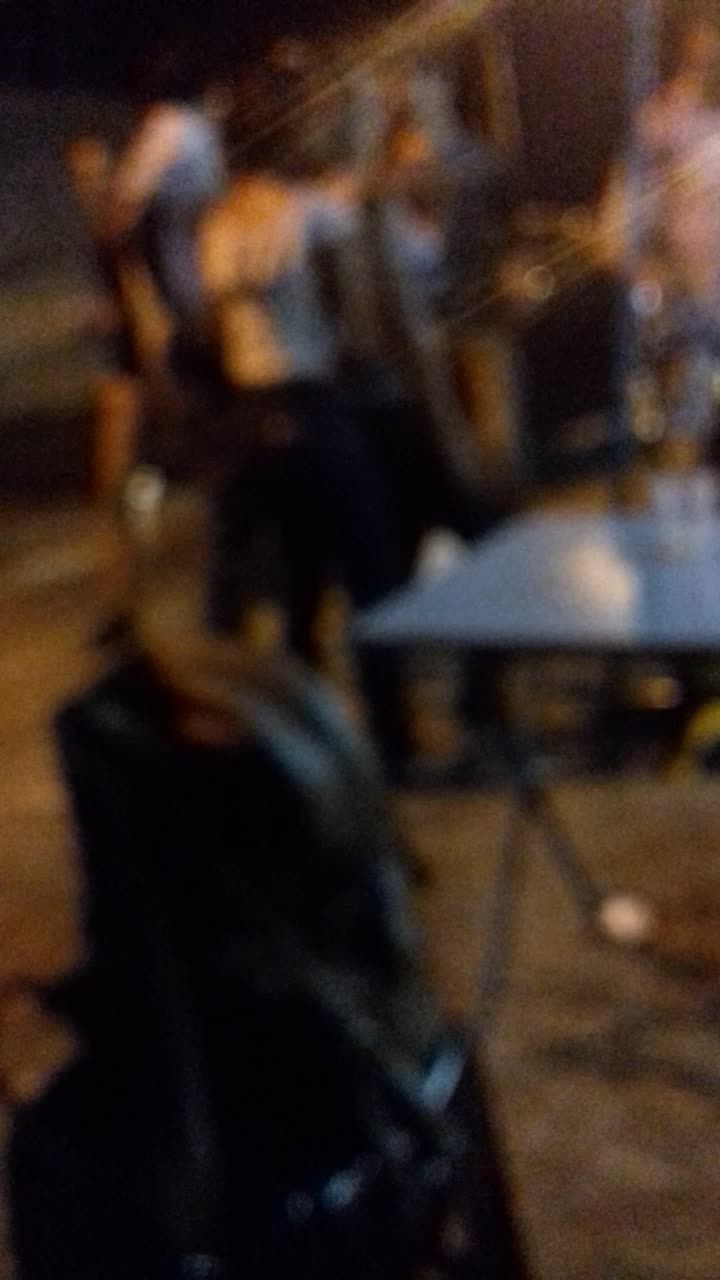In this blurred photograph taken outdoors, the most discernible element is a folding table positioned towards the middle right side of the frame. The table has a notably thin top supported by two legs that crisscross. In the background, several people can be seen standing; the first individual on the left appears to be wearing a black vest over a light-colored shirt. Next to him, another person is standing sideways, dressed in a white short-sleeved shirt. Towards the bottom of the image, there's a figure whose back is facing the camera, seemingly dressed in what resembles a Roman guard uniform. The ground appears brown, and additional figures are faintly visible amidst the indistinct backdrop.